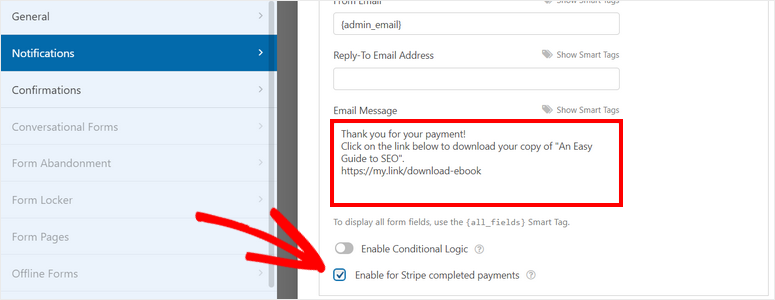Detailed Caption: 

The image is a screenshot of an email web page interface. The layout is divided into two main sections. On the left-hand side, there's a vertical navigation menu listing various options in sequence: "General," "Notifications" (highlighted in a darker blue), "Confirmations," "Conversational Forms," "Form Abandonment," "Form Locker," "Form Pages," and "Offline Forms."

On the right-hand side, there is a configuration panel with several text boxes and options. At the top, a text box labeled "Admin Email" is shown, followed by another labeled "Reply To Email Address." Adjacent to this is an option labeled "Show Smart Tips." 

Below these fields, there is another section starting with a text box for the "Email Message," also accompanied by the "Show Smart Tips" and "Tags" options. Within this text box, there is a red-highlighted message saying, "Thank you for your payment. Click on the link below to download your copy of an easy guide to SEO," followed by a clickable link.

Further down, there's an informational note stating, "To display form fields, use the [all_fields] smart tag," along with a toggle button labeled "Enable Conditional Logic," which is turned off. Additionally, there is a prominent large red arrow pointing to a checkbox option labeled "Enable for Stripe Completed Payments."

Overall, the screenshot provides a comprehensive view of the settings and configurations available on the email web page.